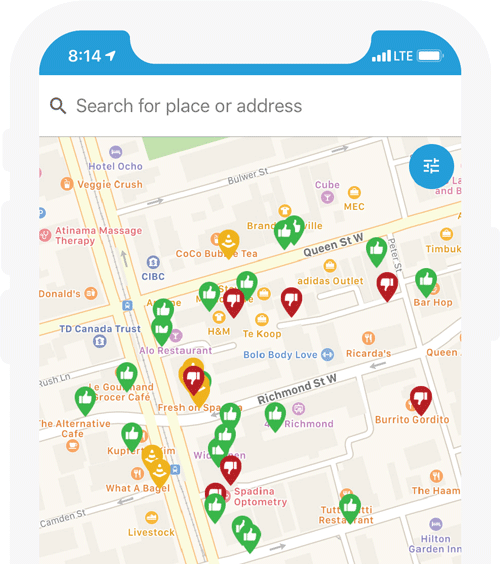A mobile screenshot depicts a directions or maps app interface. At the very top, there's a blue phone cutout outline that includes indicators for the time (8:14), full signal bars, LTE connectivity, and full battery. Below this, a white search bar with a magnifying glass icon prompts users to "search for place or address."

The map below this search bar is yellow-hued and details an area with intersecting streets: Queen Street connects to Peter Street, which, in turn, leads into Richmond Street West. A blue circle with a settings icon, reminiscent of adjustable dials, is situated in the top right corner of the map.

Various pins color the map: several green thumbs-up pins denote different restaurants or locations of interest, scattered amidst red thumbs-down pins, of which there are seven. Additionally, some yellow pins marked with traffic cone symbols suggest areas with potential construction or caution zones. Overall, the map is moderately populated with these markers against a backdrop of streets and urban layout.